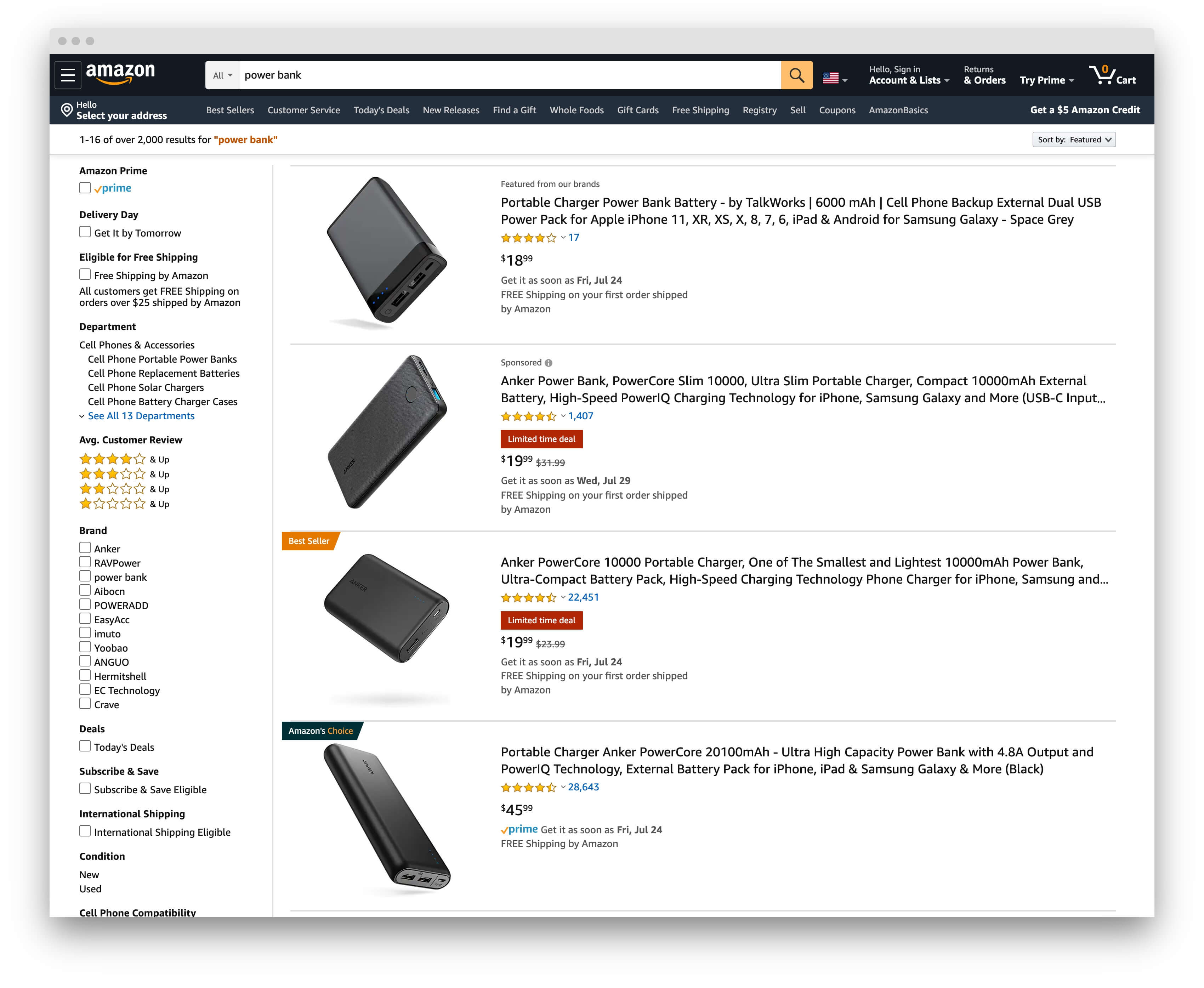The image is a detailed screenshot of a computer screen displaying the Amazon website. In the upper left-hand corner, the iconic white "Amazon" logo is prominent against a black header that spans the top of the page. To the right of the logo, there's a search bar where the term "Power Bank" has been entered. 

In the upper right corner of the screen, a shopping cart icon is visible, indicating the user's account activity. The main section of the screenshot shows the results for the search term "Power Bank," displaying four different options. Each product is depicted with an image on the left side, accompanied by detailed information on the right.

The third product down features a small orange banner in its upper left corner, designating it as a "Best Seller." Directly below, the fourth item displays a black banner that reads "Amazon's Choice," signifying it has been highlighted by Amazon for its quality and favorable reviews. 

Additionally, the second and third products have red banners over their prices, indicating that they are available at a discounted rate for a limited time only, suggesting these are time-sensitive deals. The layout and detailed elements of the screenshot highlight the various promotional labels that Amazon uses to guide consumer choices.